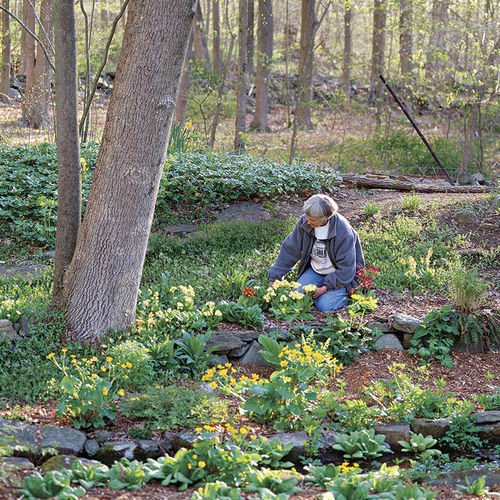The photograph captures a serene moment of an older woman, kneeling in a wooded area, attentively tending to a vibrant flowerbed. She has gray hair and is dressed in a blue jacket, white shirt, and blue jeans. Her hands are delicately working with the blossoms, which are predominantly red and yellow. To her left stands the large trunk of a tannish-colored tree, while in the foreground, further yellow flowers and various plants peek into view. A meticulously arranged rock wall and some mulch add structure to the garden bed. Behind the woman, a walking trail is visible, lined with green bushes and more trees, enhancing the tranquility and natural beauty of the scene. The overall atmosphere suggests that she has dedicated much care and effort to her gardening, creating a peaceful and picturesque setting.